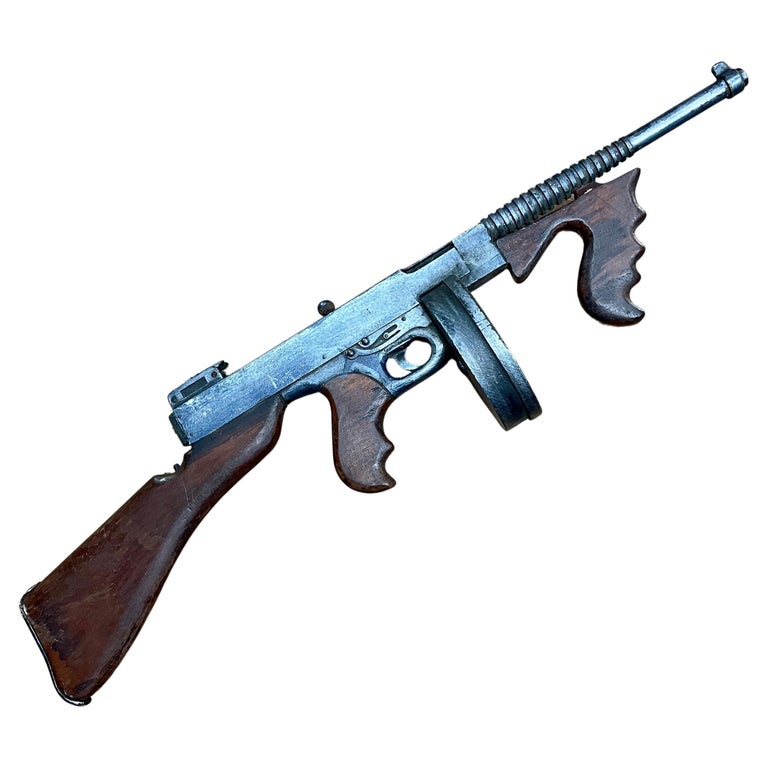The image features a Thompson M1927 submachine gun, commonly known as a Tommy gun, set against a white background. The firearm is displayed in a slanted position, with the wooden butt pointed towards the bottom left and the barrel aimed towards the top right. The gun’s body is primarily composed of silver-colored metal, while the butt, grip, and foregrip are crafted from dark wood, featuring grooves for better handling. A distinguishing characteristic of this weapon is its round, canister-like magazine situated below the barrel, indicative of the classic Tommy gun design. The barrel itself has ridges on its lower half, adding to the detailed craftsmanship of the firearm. The image is clear and brightly lit, highlighting the gun’s clean and polished appearance without any additional objects or markings in the background.